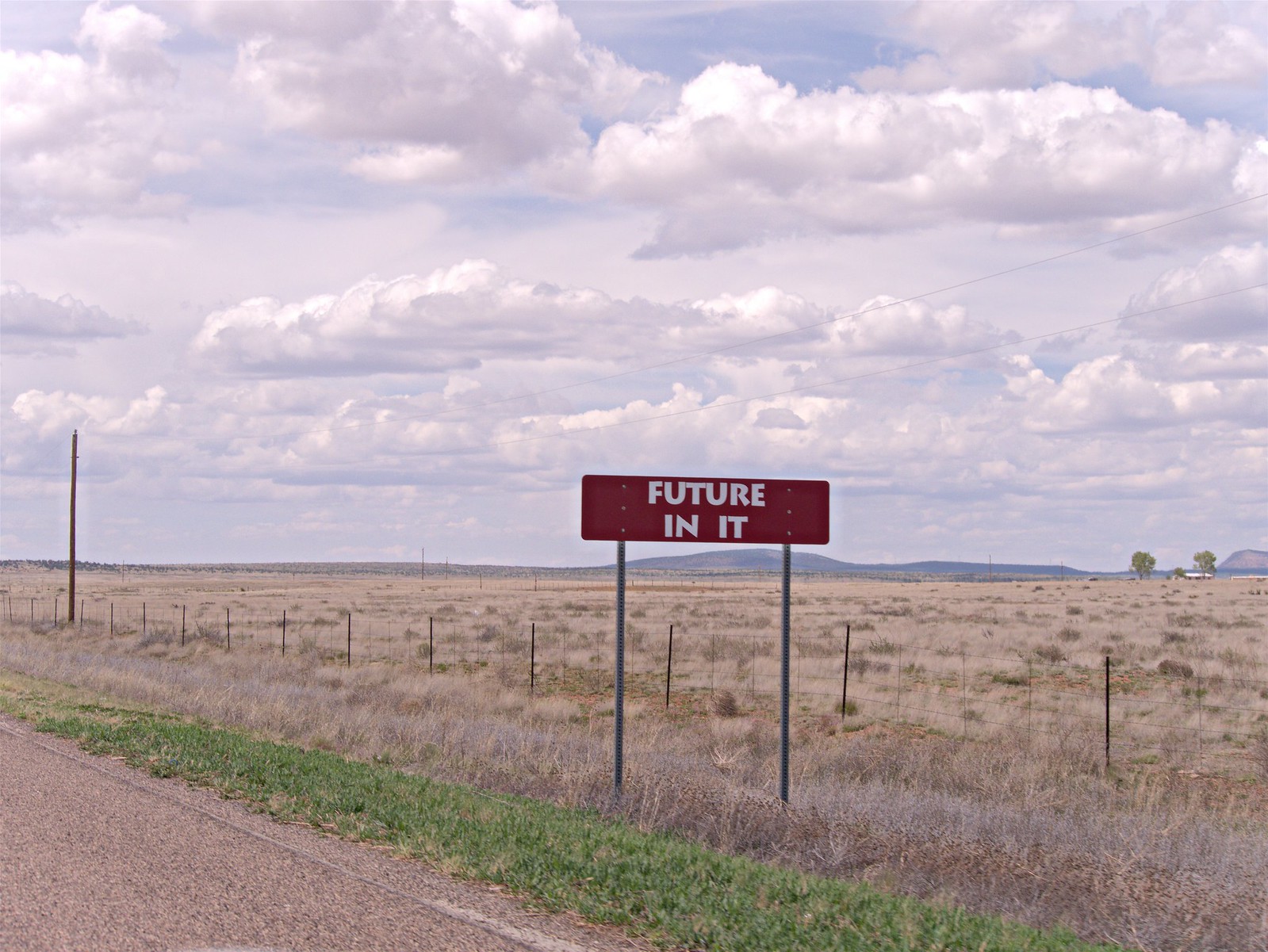The image captures a stunning landscape with a sky filled with dimensions and textures. Fluffy, voluminous clouds dominate the sky with a darker blue hue framing the tops of these clouds, while a light blue expanse below features delicate, wispy clouds. In the distance, slightly right of center, a mountain range stretches across the horizon. This range spans approximately three-quarters of the image, introducing a brief flat area adorned with two trees before another smaller mountain peaks in.

The foreground showcases a vast, flat field, likely of grain, bordered by diagonal streaks of grass at the very bottom of the image. A black-post chain link fence adds a dimensional boundary in the near view. To the far left, a solitary person stands near a road sign, contributing a contemplative human element to this serene landscape. The sign, brown with white lettering, reads "future," inviting viewers to ponder the vast expanse ahead. The individual appears to be gazing either towards the expansive field or the distant mountains, encapsulating a moment of introspection against nature's grand backdrop.